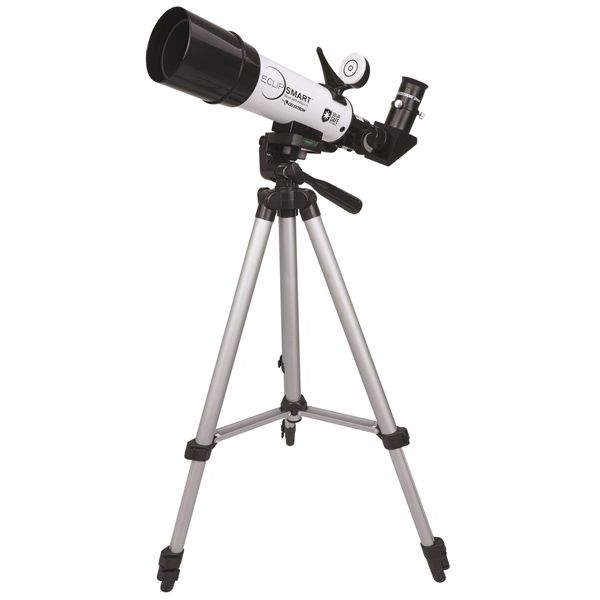The photograph features a beginner's telescope known as the Eclip Smart, designed for basic astronomical observations. The primary body of the telescope is white, accented with black components around the lens, the eyepiece, and the lever used for maneuvering it. This telescope is mounted on a silver, three-legged tripod, which includes black accents at the feet and joints. The tripod appears to be adjustable both in height and angle, enhancing user convenience. The telescope includes a sight or viewfinder on top, allowing for easier viewing without needing to crouch. The lens, though not exceedingly long, seems sufficient for casual stargazing and possibly for observing eclipses, hinted by the telescope's name and the almost full-circle design element beside the "Eclip Smart" branding. Despite being somewhat basic, this telescope appears to be functional and practical, likely within a price range of a few hundred dollars.